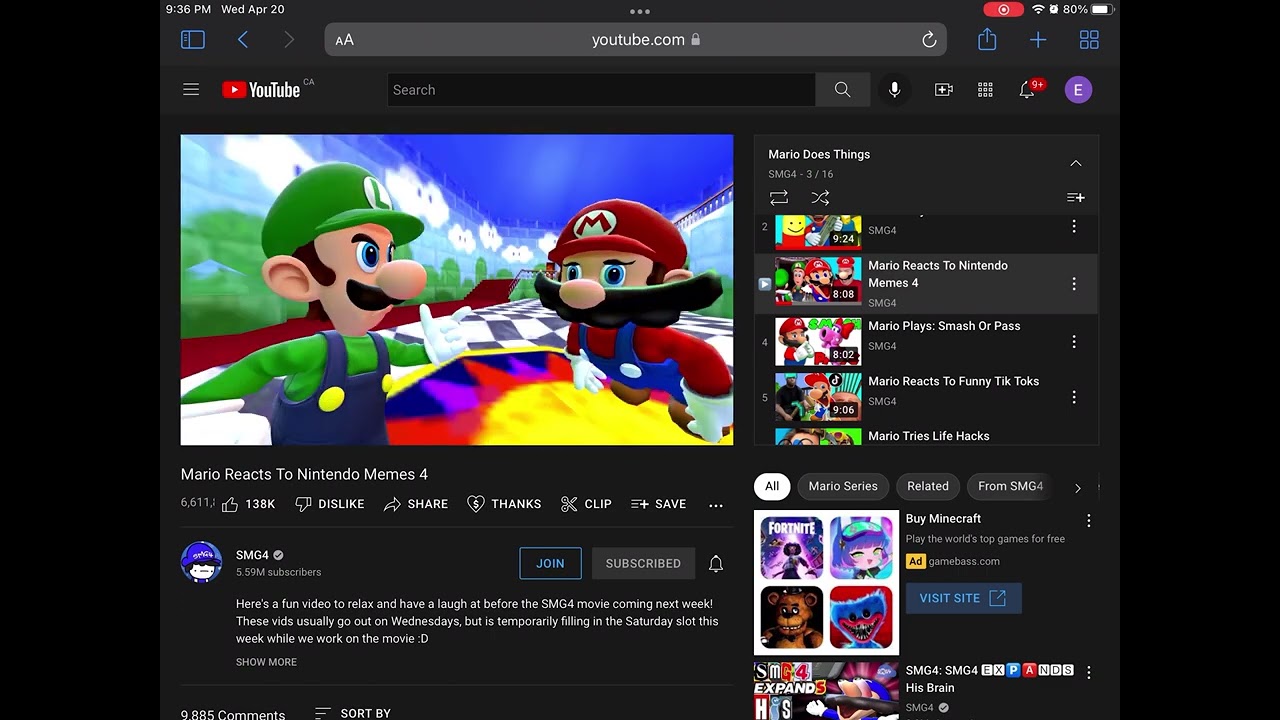Screenshot of a YouTube page showing the video titled "Mario Reacts to Nintendo Memes 4" by SMG4. The YouTube address is visible in the search bar at the top, with the YouTube logo to the left. The central focus is a still from the video featuring Mario and Luigi on what appears to be a Mario Kart-like track. Mario, sporting an unusually long mustache, is mid-jump. Luigi, with an angry expression and furrowed brow, points a finger at Mario. The background includes a painted brick wall with whimsical elements like clouds with eyes, a blue sky, and greenery. The floor has a distinctive black-and-white checkered pattern. Below the video, there is a description from the creator stating, "Here's a fun video to relax and have a laugh before the SMG4 movie coming out next week. These vids usually go out on Wednesday, but is temporarily filling in the Saturday slot this week while we work on the movie." The channel name, SMG4, is also visible.